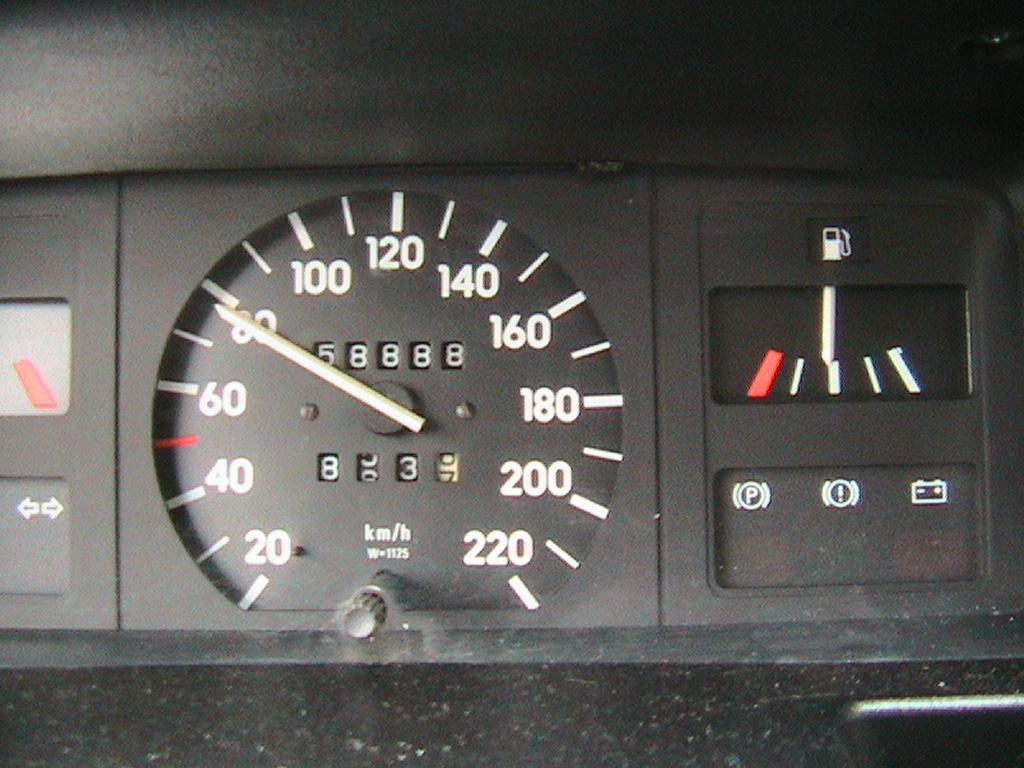Detailed image caption: 

A close-up view of a vintage vehicle dashboard, predominantly black in color, reveals an array of classic instrumentation and gauges. The older design is evident in the analog speedometer, which prominently displays numbers from 20 to 220 km/h in increments of 20. The vehicle's odometer reads 58,888 kilometers. Additionally, the trip meter shows changing digits, currently transitioning from an 8 to a 3, indicating ongoing mileage tracking.

Situated at the base of the dashboard is a small turn knob used for manual adjustments. To the right side of the dashboard, a half-full fuel gauge is visible alongside several crucial indicator symbols. These include a universal gas pump icon, a parking brake light, an unidentified warning symbol, and a battery icon, all essential for monitoring the vehicle’s status.